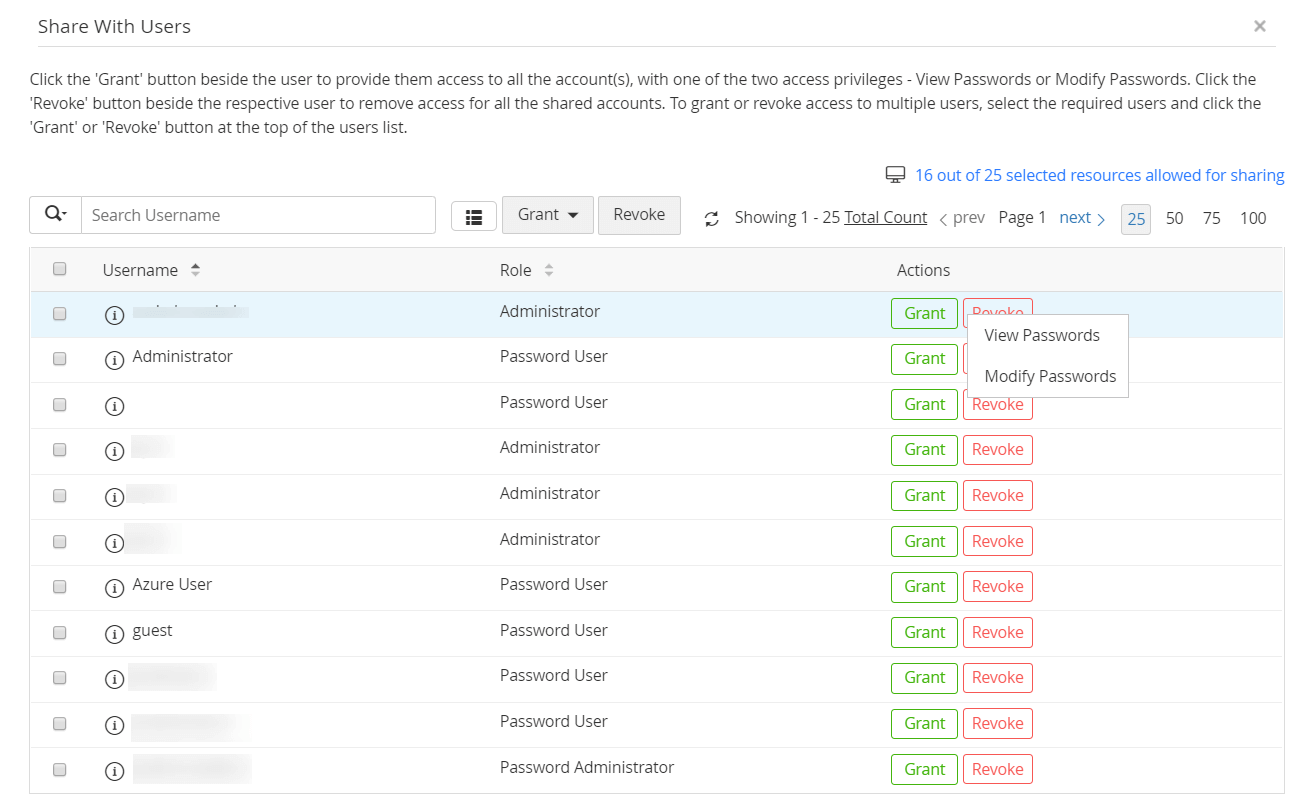The image depicts a user interface designed for managing account access privileges. The background is primarily white at the top and transitions to black on the inside. At the upper section, there's a light gray horizontal line followed by the text: "Share with users."

Beneath this line, detailed instructions in black text explain how to manage user permissions. It reads: 
- "Click the grant button beside the user to provide them access to all accounts with one of the two access privileges: View passwords or Modify passwords."
- "Click the revoke button beside the respective user to remove access for all shared accounts."
- "To grant or revoke access to multiple accounts, select the required users and click the grant or revoke button at the top of the users list."

The user list follows, with some user names blurred. The visible entries include "administrator" and "guest" among others that are similarly hidden. Each user is listed along with their respective role, indicated in a column labeled "Role." The roles vary, with labels such as "Administrator" and "Password User."

The interface also contains an "Actions" column, where each entry has two buttons: a green-outlined "Grant" button and a red-outlined "Revoke" button.

Additionally, a light gray box tab is visible over the first three rows. Within this box, in black text, are the options "View passwords" and "Modify passwords."